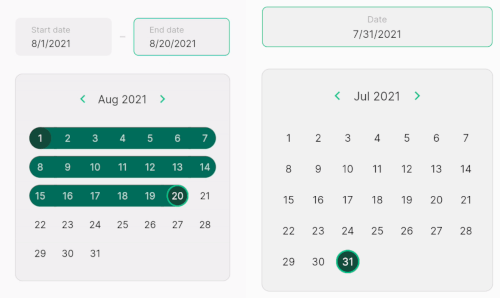The image contains two distinct screenshots of calendars placed side by side. The calendar on the left displays the month of August 2021, while the calendar on the right shows the month of July 2021. For the August calendar, there are two labeled boxes at the top: "Start Date: 8-1-2021" and "End Date: 8-20-2021." The dates from August 1st to August 20th are highlighted in green, creating a continuous block covering three weeks. Specifically, the first week includes August 1st to 7th, the second week covers August 8th to 14th, and the third week spans from Sunday, August 15th to Friday, August 20th.

In contrast, the July calendar has a single box at the top labeled "Date: 7-31-2021." Here, only one date is highlighted in green, which is Saturday, July 31st. This juxtaposition of the two calendars illustrates different periods of significance, with the August 2021 calendar highlighting a nearly three-week span and the July 2021 calendar emphasizing just a single day.